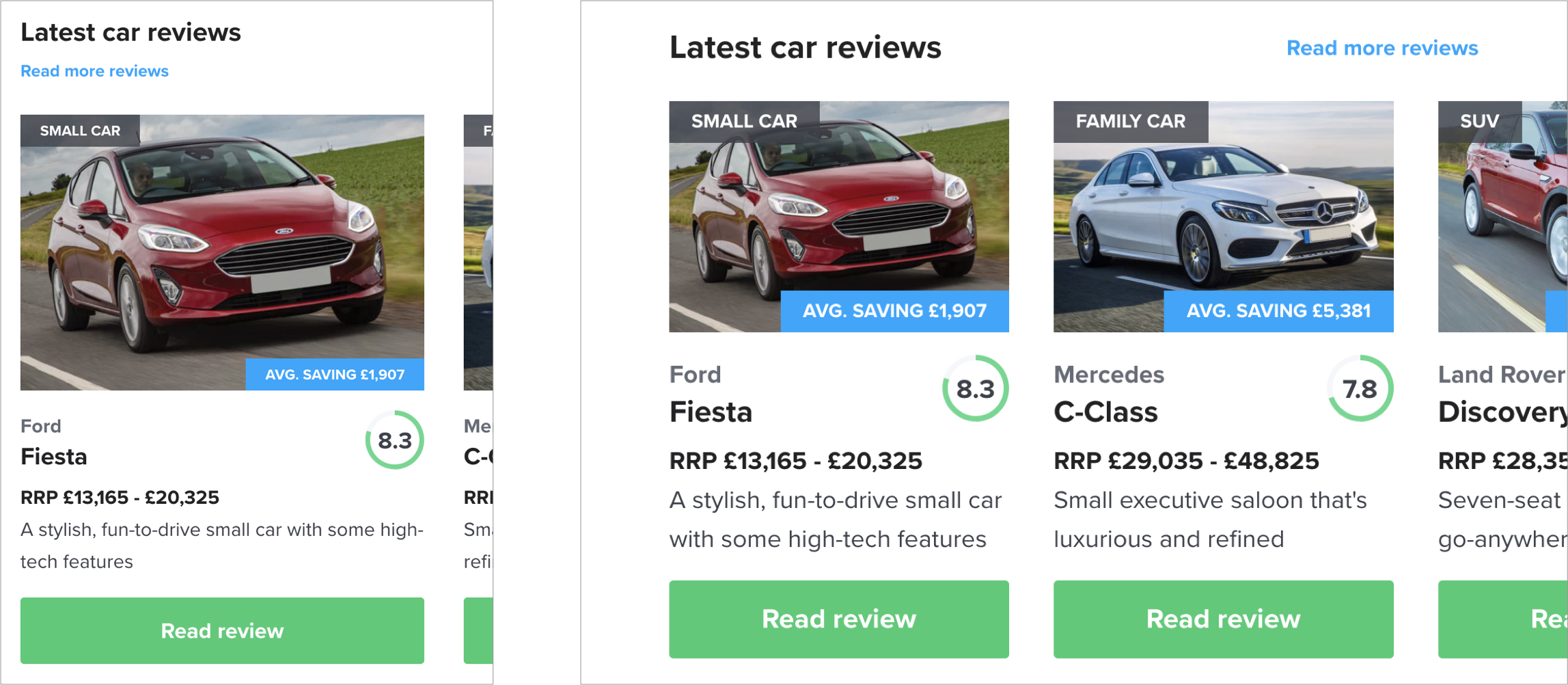This image presents a comparison layout for the latest car reviews, showcasing three different vehicles along with their respective details. 

1. **Ford Fiesta**: 
   - **Category**: Small Car
   - **Price Range**: £13,165 to £20,325
   - **Description**: A stylish, fun-to-drive small car equipped with high-tech features.
   - **Savings**: £1,907
   - **User Rating**: 8.3

2. **Mercedes C-Class**: 
   - **Category**: Family Car (Small Executive Saloon)
   - **Price Range**: £29,035 to £48,825
   - **Description**: A luxurious and refined small executive saloon.
   - **Savings**: £5,381
   - **User Rating**: 7.8

3. **Land Rover Discovery**: 
   - **Category**: SUV
   - **Price Range**: Starts at £28,035 (exact upper range is cut off)
   - **Description**: A versatile seven-seat, go-anywhere SUV.
   - **Savings**: Not mentioned
   - **User Rating**: Not shown

The layout is designed to be user-friendly, presenting key details such as car category, average savings, price range, a brief description, and a user rating for each vehicle. Additionally, each car listing includes a green "Read Review" button for further details.